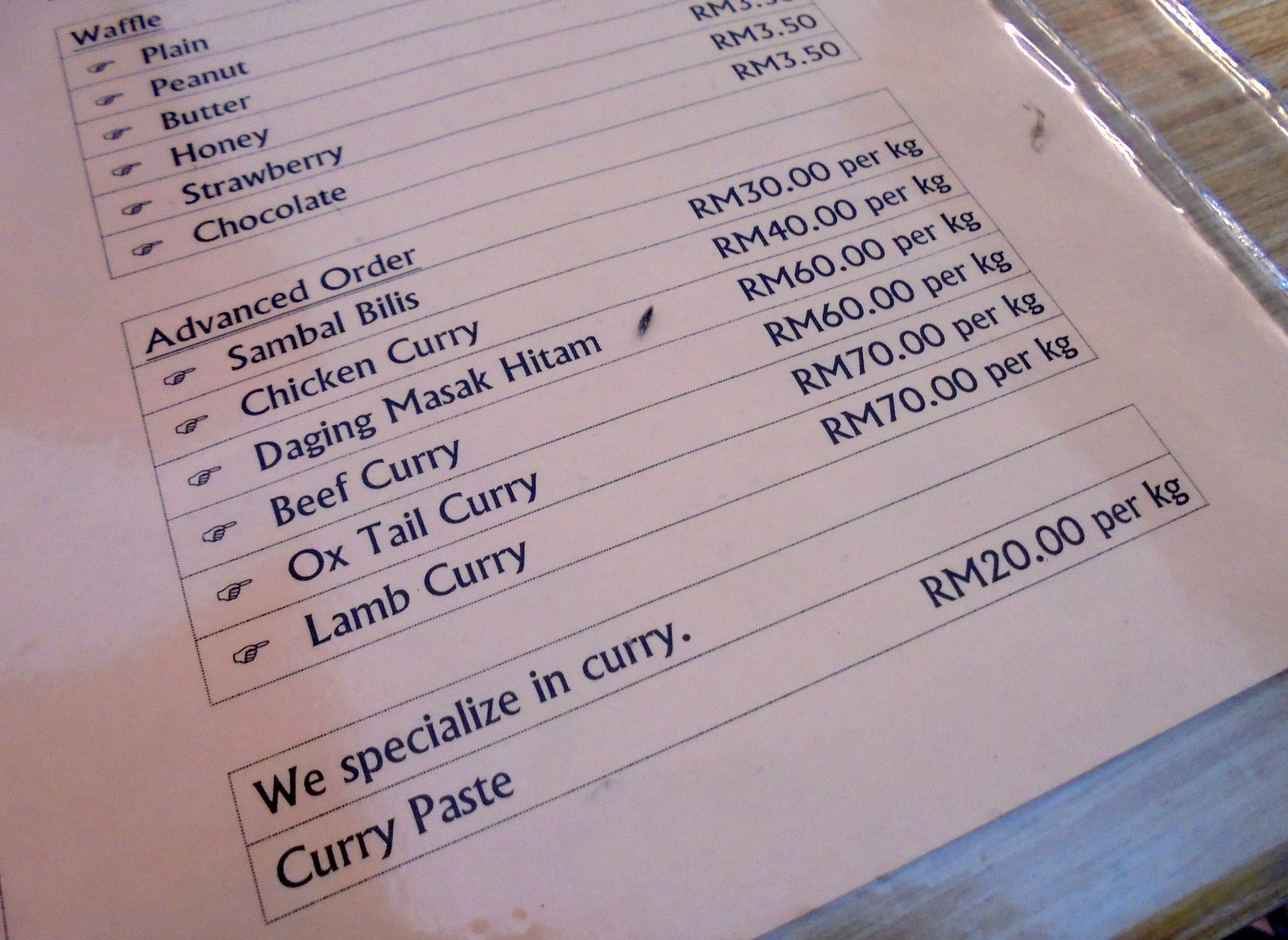This photograph depicts a laminated menu laying diagonally on a light-colored wooden table, occupying most of the frame. The menu is printed with black text on a pinkish paper, organized into two main sections. The first section, titled "Waffle", lists various waffle options such as plain, peanut, butter, honey, strawberry, and chocolate. The second section, labeled "Advanced Order”, includes more elaborate dishes like sambal bilis (RM 30.00 per kilogram), chicken curry (RM 40.00 per kilogram), daijing masa ketam (RM 60.00 per kilogram), beef curry (RM 60.00 per kilogram), oxtail curry (RM 70.00 per kilogram), and lamb curry (RM 70.00 per kilogram). Below these sections, a smaller segment mentions, "We specialize in curry, curry paste (RM 20.00 per kilogram)." The menu appears to be from an establishment that emphasizes its curry offerings, possibly an Indian restaurant.